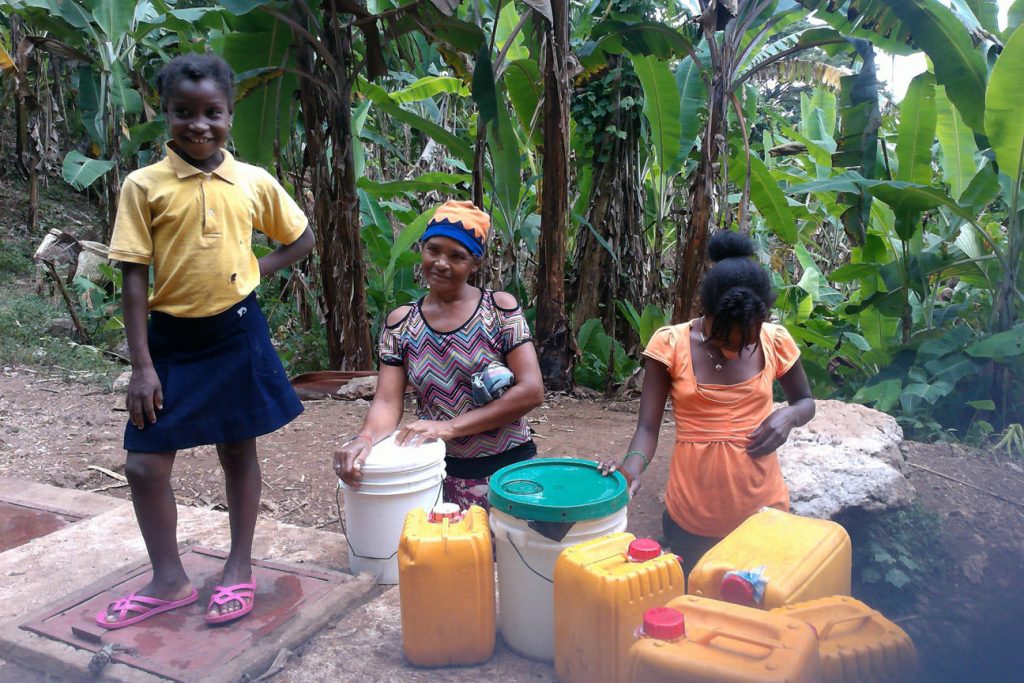In a lush, tropical forest abundant with vibrant green foliage and palm-like trees, three young black girls are gathered on a cleared dirt path with scattered wood debris. The girl on the left is standing confidently on what appears to be a metal door or access hatch leading into a cemented area. She wears a yellow polo shirt, a blue skirt, and pink sandals, her short black hair framing her smiling face.

To her right, a girl kneels on the ground, her hands resting on a white bucket with a blue lid. She wears a striking multicolored shirt with diagonal stripes and shoulder cutouts, a blue and yellow hat adorning her head. Her friendly gaze and smile are captured as she appears ready to lift the bucket's lid.

The third girl kneels beside her, wearing an orange top, dark pants, and a gold necklace. Her black hair is styled in a bun with bangs, and she looks down thoughtfully, perhaps blowing a bubble. Before her are several large yellow canisters with red lids, and another white bucket with a teal lid, neatly arranged on the ground. This serene moment captures their simple, joyful existence amidst the vibrant, natural beauty of their surroundings.